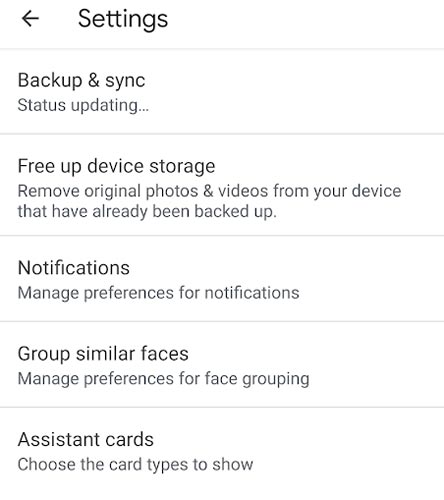In the screenshot of the settings menu, the top section showcases a left arrow icon followed by the word "Settings" in bold. Directly beneath this header, the text reads "Backup and sync status updating." 

The next row features the option to "Free up device storage" with a description underneath: "Remove original photos and videos from your device that have already been backed up." 

Following this, a row labeled "Notifications" allows users to manage preferences for notifications.

The subsequent row, titled "Group similar faces," offers settings to manage preferences for face grouping.

The final row, "Assist cards," provides the option to choose which card types to display.

All the text is rendered in black font against a white background. Thin light gray lines separate each row, creating a clear division between the different settings options.